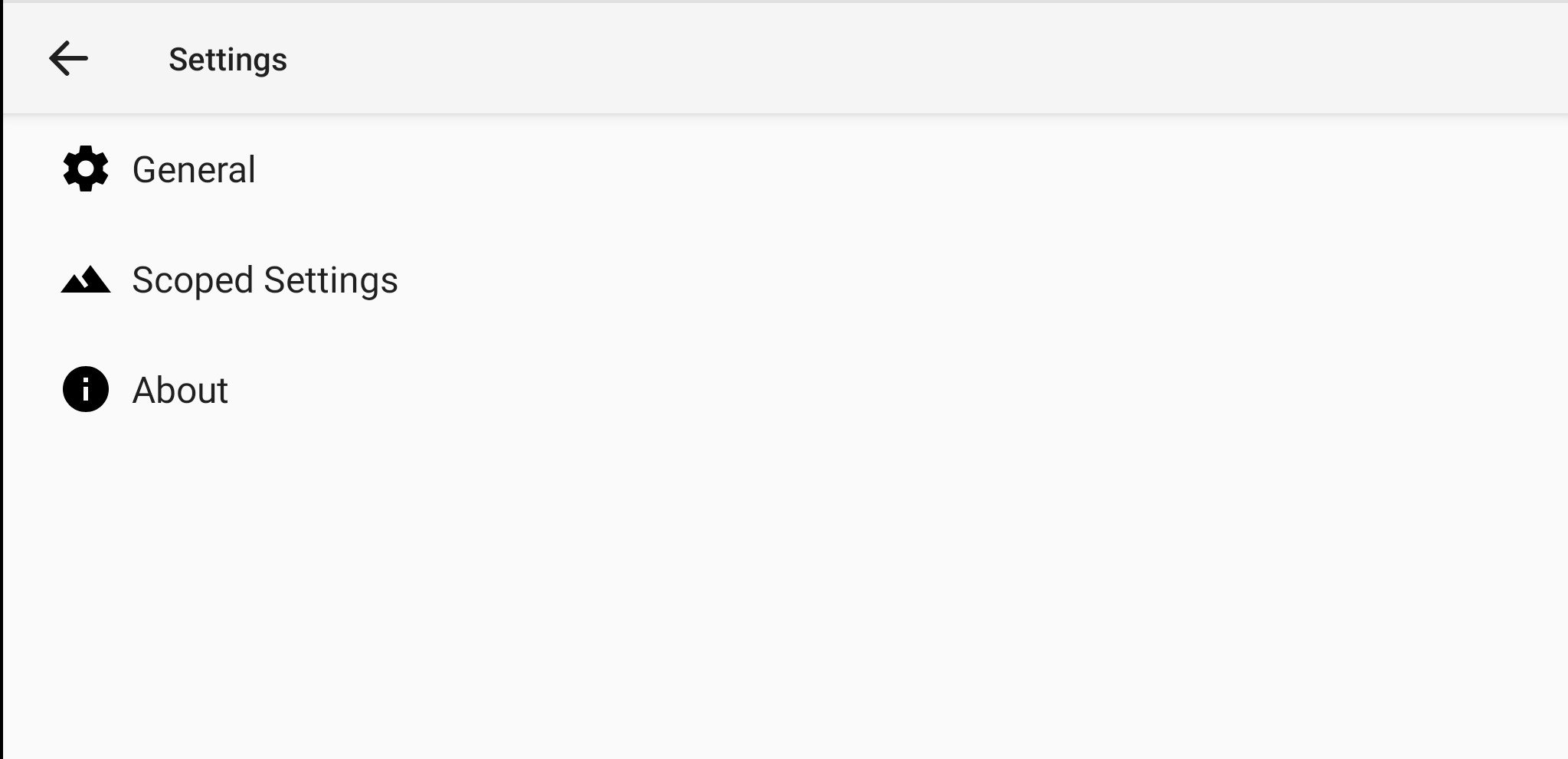The image displays the settings interface of a website, characterized by a minimalist design featuring grey and black tones. At the top, a heading labeled "Settings" is accompanied by a leftward-pointing arrow. Below this heading, the menu includes three primary sections: 

1. "General" is preceded by an icon resembling machinery or gears.
2. "Scope Settings" is marked by a symbol resembling a mountain with a missing segment.
3. "About" features an icon depicting an eye enclosed within a circle.

The background predominantly consists of a light grey hue, with a slightly darker grey highlighting the active "Settings" tab. A bold black line delineates the left side of the menu. The icons are rendered in solid black, while the text appears in a lighter black or very dark grey, presented in a simple font likely to be Arial or Calibri. The menu bar where "Settings" is mentioned has a shading effect beneath it, adding subtle depth. The right side of the image remains largely vacant, punctuated only by the grey border and shading around the settings tab. Overall, the design is clean, with ample empty space on the right side of the image.